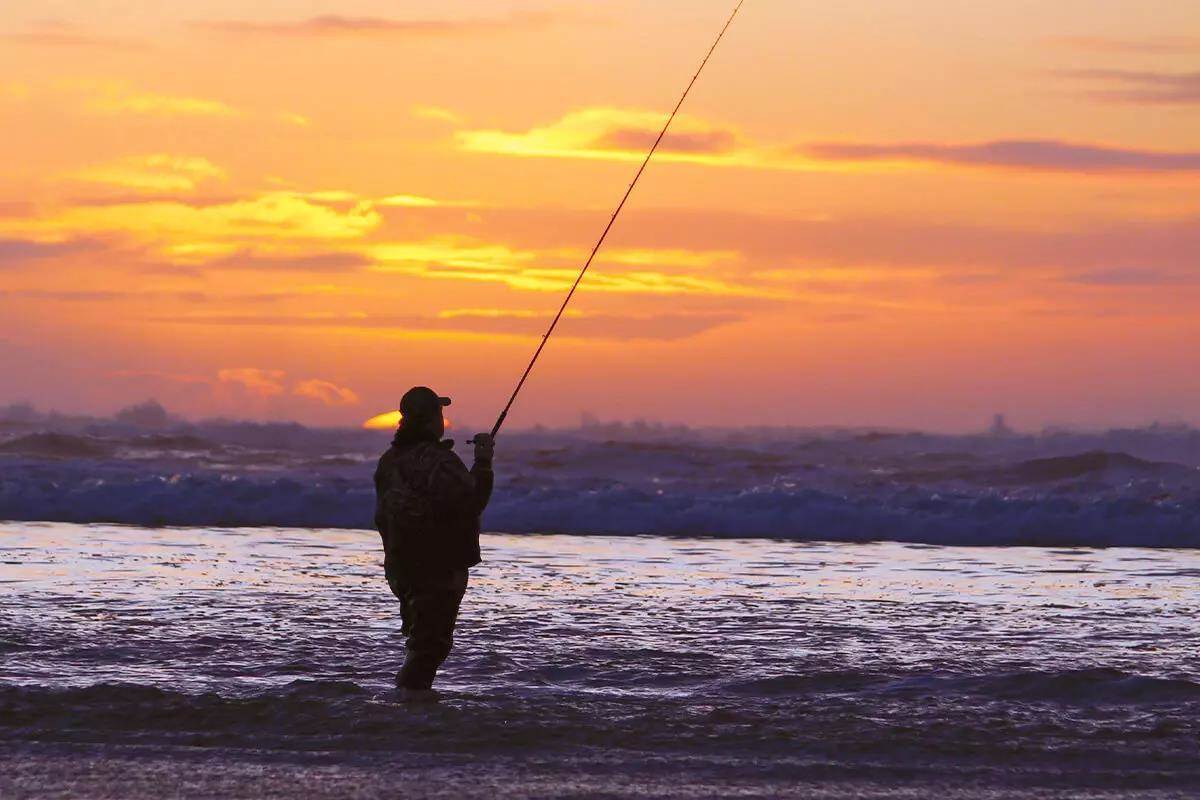The photograph captures a silhouetted man standing ankle-deep at the shore of a body of water, engaged in fishing. The scene is bathed in the stunning orange and yellow hues of either sunrise or sunset, with the very top of the sun just peeking over the horizon. The sky is a mesmerizing blend of orangish-red with yellow-tinged clouds, casting a serene glow over the landscape. The water around him ripples with waves that reflect the colors of the sky. The man, whose features are darkened and obscured by the low light, is clad in a heavy coat, long sleeves, and pants, and he wears a hat. He holds a very long fishing rod that extends from his hand towards the top of the image, though the fishing line itself is not visible. In the distant blurry background, some buildings can be seen, adding a minimal yet notable detail to the tranquil setting. The overall atmosphere exudes a sense of peaceful solitude and connection with nature.